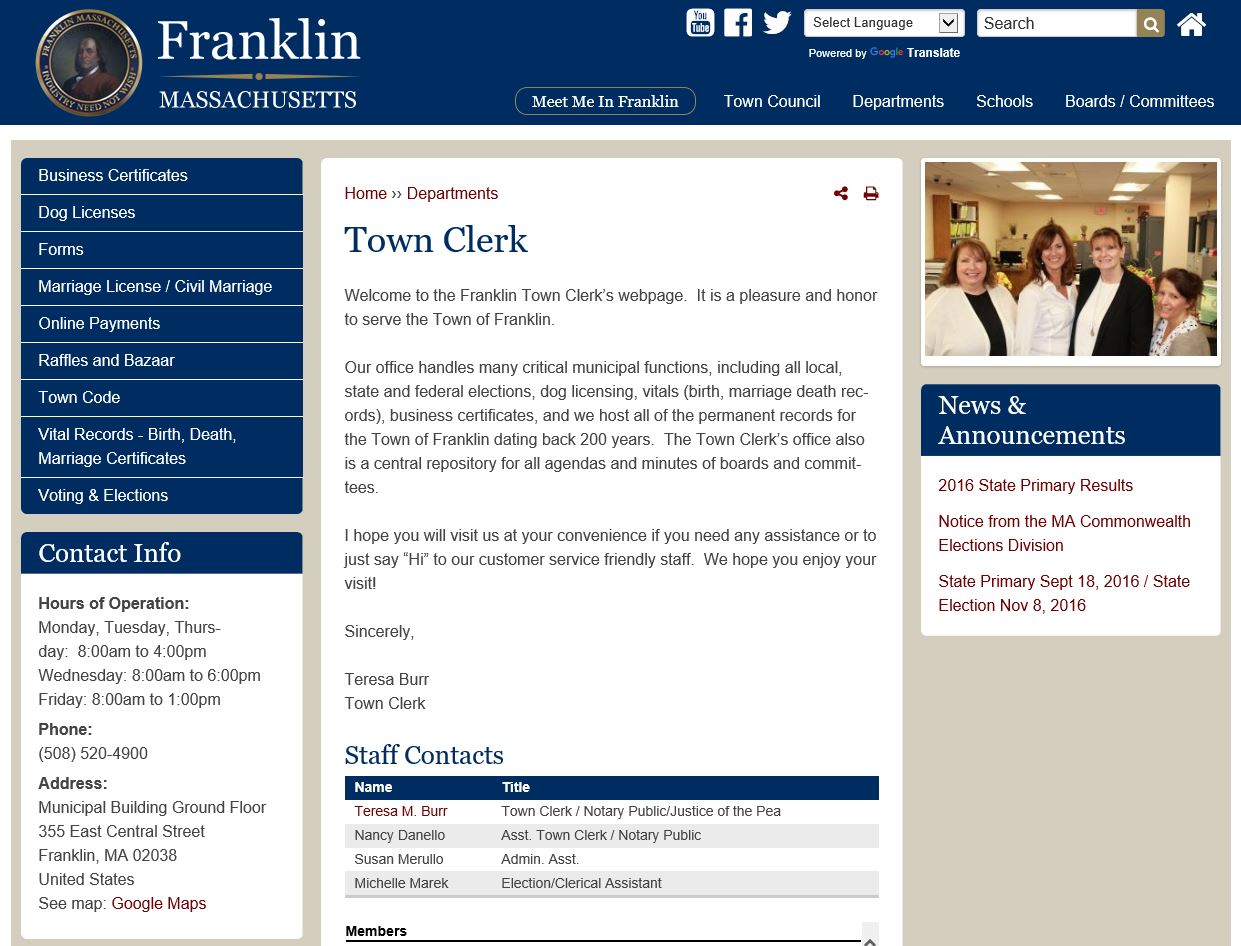Screenshot of the official website for Franklin, Massachusetts.

At the very top of the webpage is a prominent blue navigation bar featuring essential information and tabs. On the left side of the bar, the text "Franklin, Massachusetts" is displayed next to a round image of a man, encapsulated within a circular frame. Beneath the image, the town's motto, "Industry Need Not Wish," is inscribed. 

The navigation bar includes five tabs, labeled: "Meet Me in Franklin," "Town Council," "Departments," "Schools," and "Boards/Committees." On the right side of the bar, users can find contact information, social media icons, a language selection drop-down, a search bar, and a home symbol.

Below the navigation bar, in the central portion of the webpage, is an article titled "Town Clerk." This section contains a welcome message and essential information about the Town Clerk's office. At the bottom of this article, there is a list of staff contacts, including their names and titles.

On the left side of the webpage is a sidebar with various categories for easy navigation: "Certificates," "Dog Licenses," "Forms," "Marriage License/Solo Marriage," "Online Payments," "Raffles and Bazaar," "Town Code," "Vital Records," "Voting and Elections," and "Contact Info."

On the right side of the page, there is a "News and Announcements" section featuring links to recent updates and news. Just below the top navigation bar, on the right, an image of four Caucasian women, who are presumably members of the Town Clerk's office, is displayed.

This detailed layout ensures residents and visitors can easily access information and resources related to Franklin, Massachusetts.